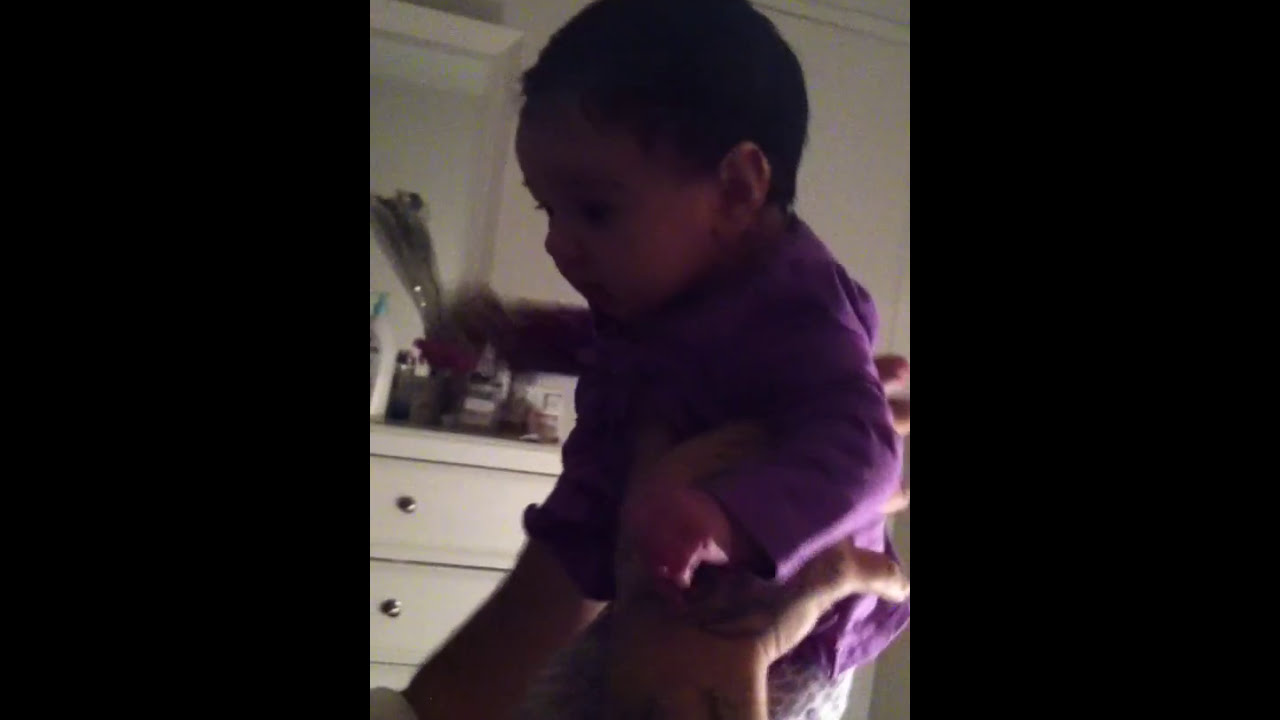The image features a dimly lit, slightly grainy photograph with vertical black borders along the left and right sides. At the center, an individual, only their arms visible, is holding up a very young child. The person has a wristwatch on their left hand. The baby, who has short, dark hair, is facing left with a calm, content expression and is dressed in a purple shirt and patterned white and purple pants. The background reveals a white wall and a white dresser to the left. The dresser has a top mirror or frame and is adorned with various items, including jars, bottles, and a white lotion bottle. The light source seems to be closer to the ground, partially illuminating the scene, suggesting the photograph might have been taken in a child's room, possibly for social media.